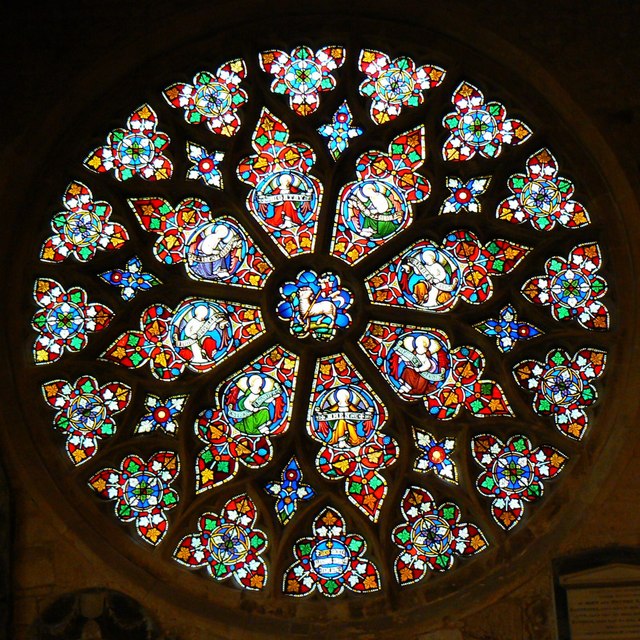The image depicts a meticulously detailed, color photograph of a circular stained glass window, commonly known as a rose window. It is set against a dark, night sky, providing a stark contrast that enhances its vibrant colors. The photograph is taken from a vantage point looking directly upward, capturing the window in its entirety.

The rose window features an intricate, multi-layered design. The innermost section is adorned with a figure of a sheep set against a blue sky background. Surrounding this central figure are eight tapered, petal-like sections, each containing unique, elliptical illustrations of individual figures. These characters are depicted in varied robes of green, orange, and red, each engaged in different symbolic actions. Notably, one figure in a red robe holds a banner, while another in green appears to cradle a scroll in its lap.

Encompassing these petals is an outer layer with cross-shaped stained-glass elements placed between each petal section. This band further extends into a border of triangular stained glass pieces in an array of different colors, culminating in an elaborate butterfly design where no two butterflies are identical in position or coloration.

The overall photographic style is rooted in representational realism, capturing the minute details and the architectural complexities of the stained glass window, which appears to be situated atop an arch structure partially visible at the bottom left and right of the frame. The image depicts the artwork with a sense of awe and clarity, highlighting the craftsmanship and artistic diversity of the stained glass medium.